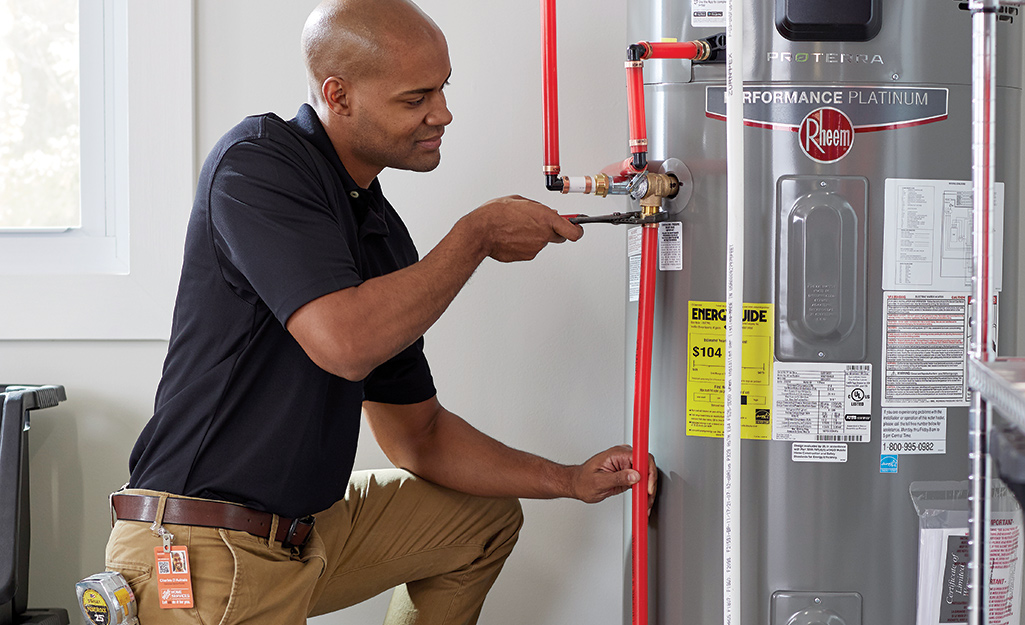The image shows an African-American technician, characterized by his brown skin, working meticulously on a clean, large water heater that is likely a 55 or even an 80-gallon unit. The water heater bears several labels, including a prominent bright yellow energy guide sticker and the Performance Platinum label from the Rheem brand. He is wearing a dark blue or black polo shirt tucked into dark khaki pants, with a belt holding an identity badge and a measuring tape. The technician is positioned in a garage or a white-walled room with a window to the left. He is either kneeling or has one leg lifted, with his left elbow resting on his knee as he uses a wrench to tighten an orange pipe connected to the water heater's complex network of red, bronze, and other colored tubes. His clean and professional appearance, along with his clear and deliberate pose, strongly suggests that this image is designed as an advertisement for a company specializing in water heater installation or repair services.